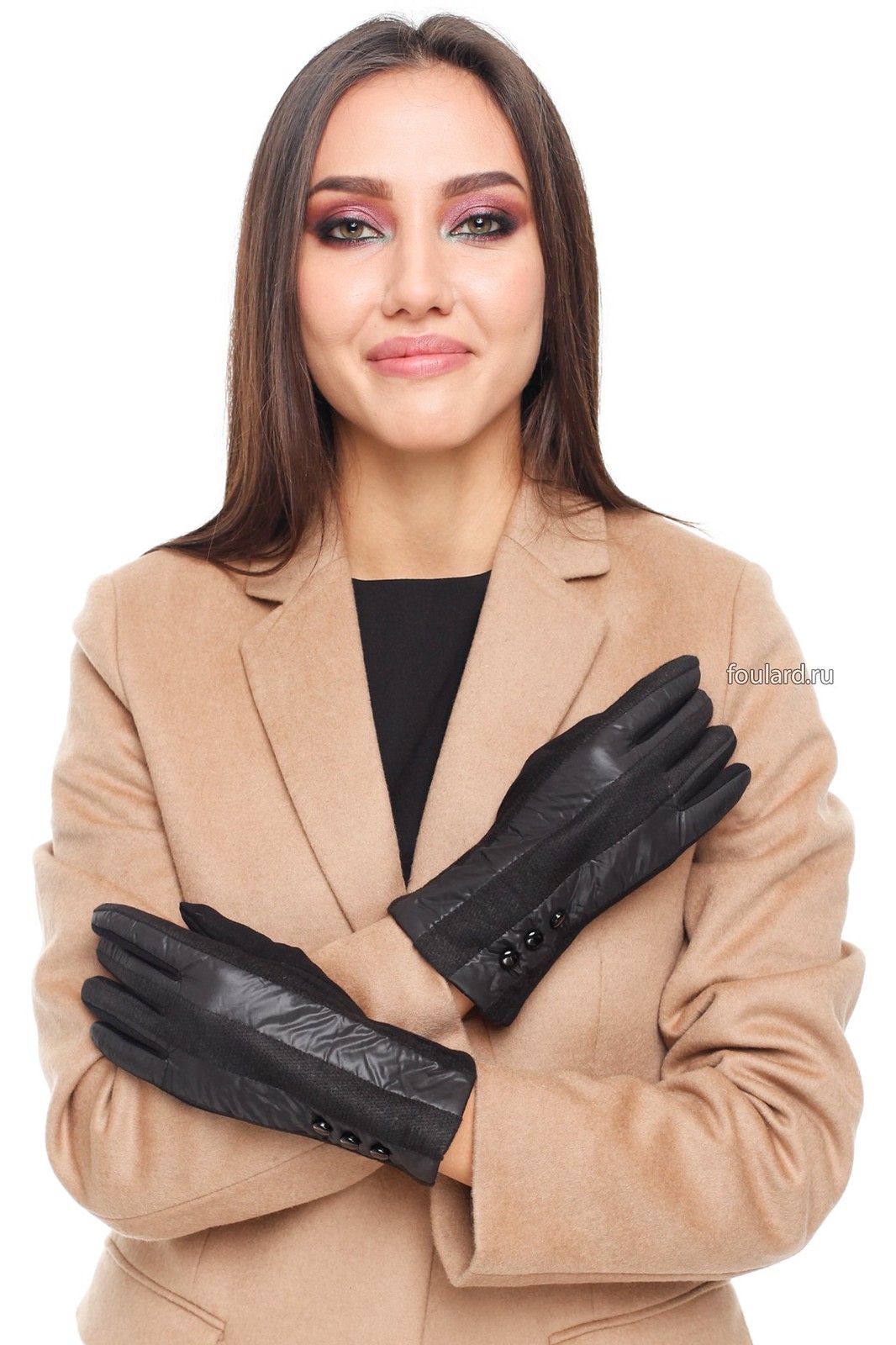The photograph is a professional studio shot, showcasing a woman who appears to be modeling for a fashion advertisement. The background is a perfect, crisp white, emphasizing the clarity and quality of the image. Labeled in a digital font over her right shoulder, the text "foulard.ru" likely indicates the website URL for the business being advertised.

The model has shoulder-length, dark brown hair that falls past her shoulders and down her back, parted in the middle. She is wearing heavy makeup, including red and purple eyeshadow, heavily shaded black eyeliner, and pink lipstick. She gazes directly at the camera with a slight, closed-mouth smile, her eyes large and slightly narrowed, giving her an enigmatic expression.

She is dressed in a tan or beige blazer that extends out of the frame at her waist, with a black round-neck top or T-shirt underneath. Her arms are loosely crossed in front of her, with the left arm below and in front of the right arm, which is angled upwards at 45 degrees. She is accentuating a pair of black leather gloves, each adorned with three black buttons near the wrist and a central stripe of different material running down the middle. Her fingers are slightly curled as she hugs her arms to her body, drawing attention to the details of the gloves.